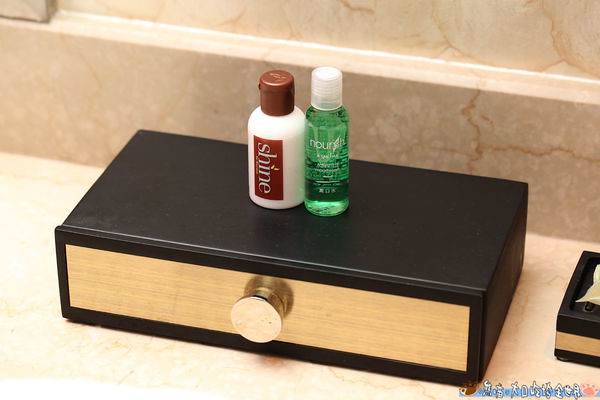The image showcases a narrow black box, reminiscent of a jewelry case, with a thick, round gold knob at the front. The frontal view highlights the gold drawer that slides out from the black exterior, which appears to have a yellowish leather texture. Inside the drawer is a small sample-sized product labeled "nourish," and another smaller sample labeled "shine," which contains white liquid and features a tan brown top complementing the label. The backdrop is either granite or marble, adding a sophisticated touch. Adjacent to the black box is another black and gold box, differently shaped and adorned with a bow. This setup is likely on a vanity, possibly in a bathroom, though the exact location is unclear due to the high wall and partial view. In the upper left corner, there appears to be a small square object, possibly a bracket or door frame.